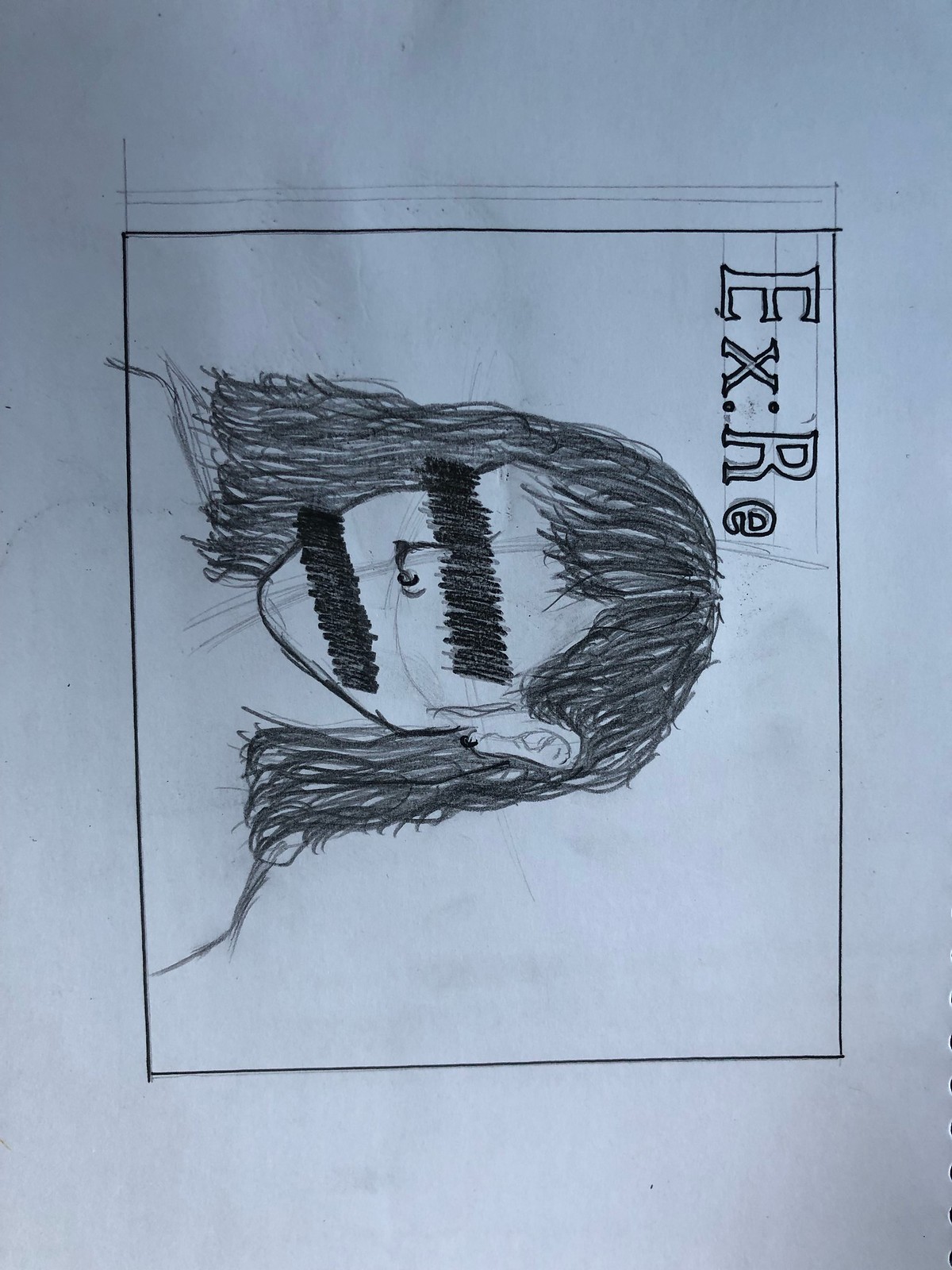The image is a sideways photograph of a pencil and marker drawing. The drawing features a person with shoulder-length dark hair, neatly cut in a blunt style with shaggy bangs across the forehead. The individual's face has been obscured by thick, black, squiggly lines, forming rectangular bars over the eyes and mouth, which completely cover these features. The person appears to be unclothed, and their shoulders are visible. The image is on a white piece of paper and is contained within a small square. The top right of the square, when viewed correctly, contains the title "Ex::Re" written in precise, capitalized letters with some lines penciled in for guidance. Additional pencil sketch lines cross through the drawing, intersecting notably at the nose and chin, adding to the abstract nature of the artwork.